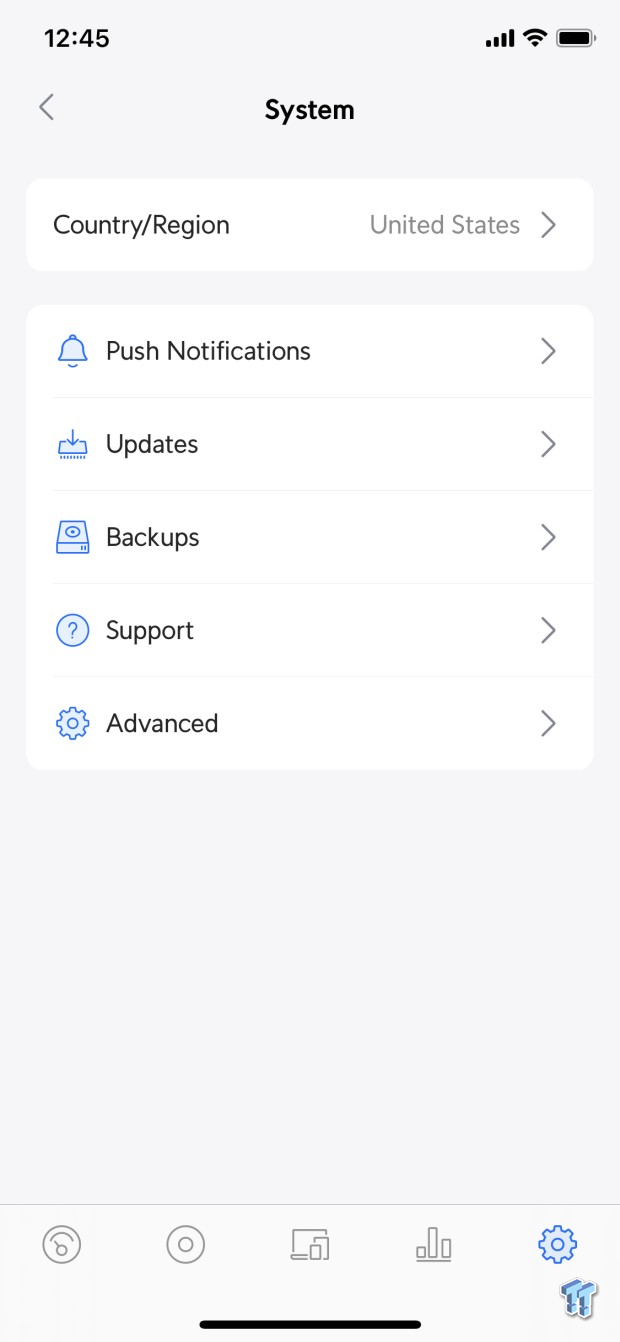The image displays a webpage on an iPhone. In the top-right corner, the battery icon is fully charged, and the signal strength is at maximum with four bars. The time shown is 12:40. At the top of the webpage, the word "System" is written in black lettering with a left-pointing arrow beside it. Below this header is a long, white, rounded-edged box labeled "Country/Region" with "United States" written inside and a right-pointing arrow.

Beneath this section are several white boxes with various options:
1. "Push Notifications" - represented by a blue bell icon with a right-pointing arrow.
2. "Updates" - indicated by a blue icon resembling a flat box with a downward arrow, also accompanied by a right-pointing arrow.
3. "Backups" - depicted with a box and a circle on top, giving it a 3D effect, and a right-pointing arrow.
4. "Support" - shown as a blue box with a question mark in the center and a right-pointing arrow.
5. "Advanced" - marked by a blue settings gear icon and a right-pointing arrow.

The background below these options is gray, typical of the iPhone interface. At the bottom of the screen, there are various icons including a pair of side-by-side, inverted L-shaped symbols in the lower-right corner.